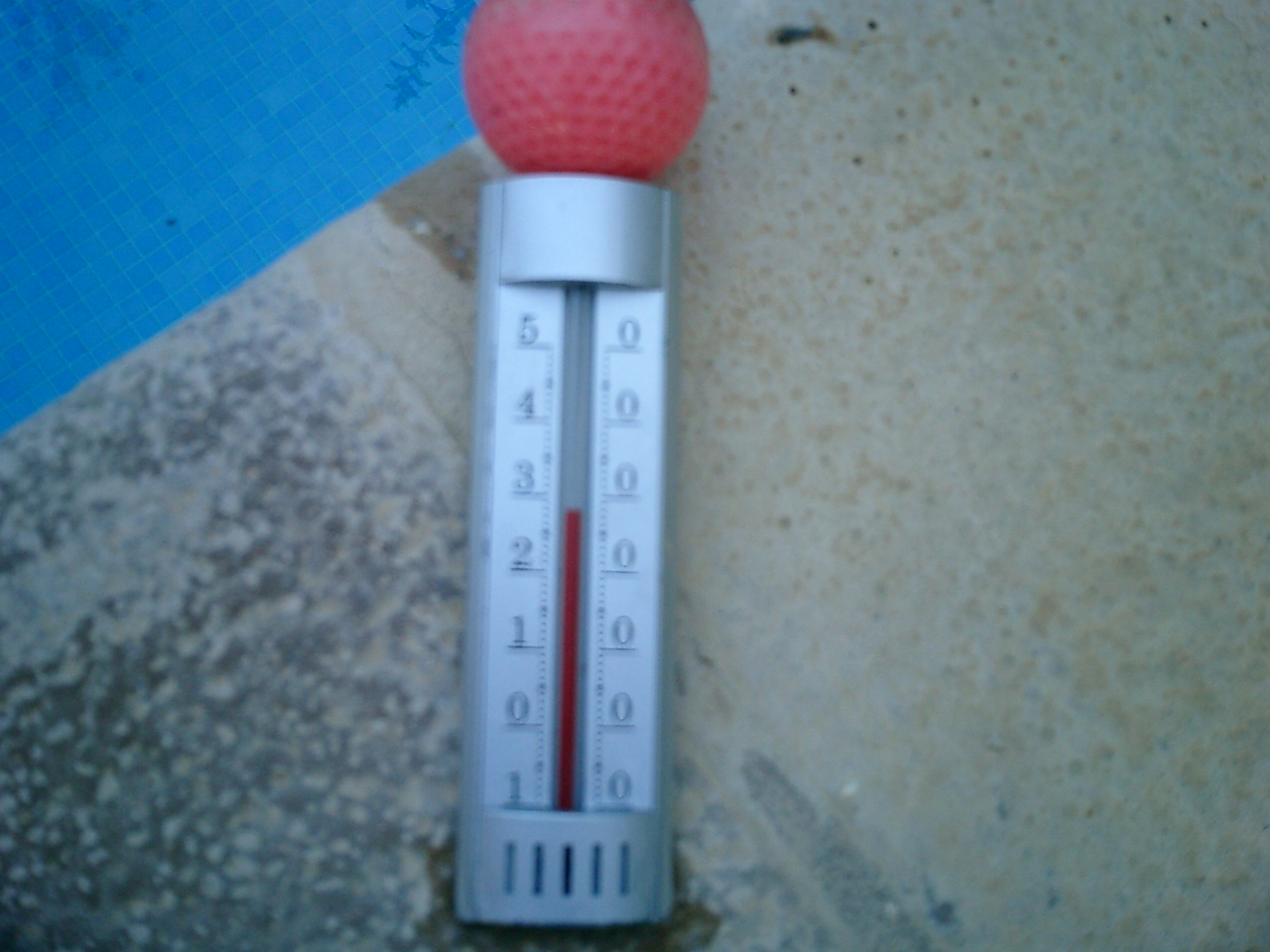A close-up, unfocused photograph captures a water temperature meter placed on a light beige concrete surface next to a pool. The pool, occupying the top left corner of the image, features blue tiles and shimmering water, with shadows of nearby trees gently reflecting on its surface. The concrete dominates approximately 80% of the photograph. The centerpiece is a silver temperature meter adorned with a hollow red golf ball on top, designed to float and indicate water temperature. The meter's left side is marked with numbers from 0 to 5, while the right side displays zeros. The red indicator on the meter shows a temperature reading hovering closer to 3.